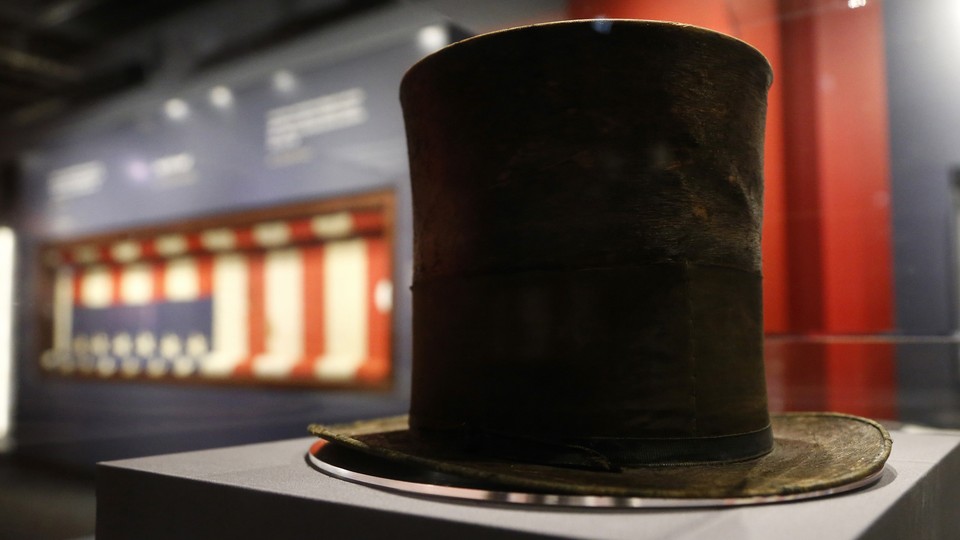The image features a tall, dark top hat with a brown brim, reminiscent of a magician's hat and possibly made of a thick, corduroy-like material. The hat is placed on a reflective pedestal or table. In the background, there is a partially rolled-up American flag with visible stars, blue sections, and red and white stripes. This flag is part of a black display area, with a noticeable red column situated directly behind the hat. Additionally, there is a light in the top right corner illuminating the hat, causing the upper part to appear darker and less visible. The overall scene evokes a sense of nostalgia, similar to the iconic top hat worn by Slash from Guns N' Roses, accentuated by the mysterious, potentially jukebox-like structure with its glass dome and lit-up red and white accents in the background.